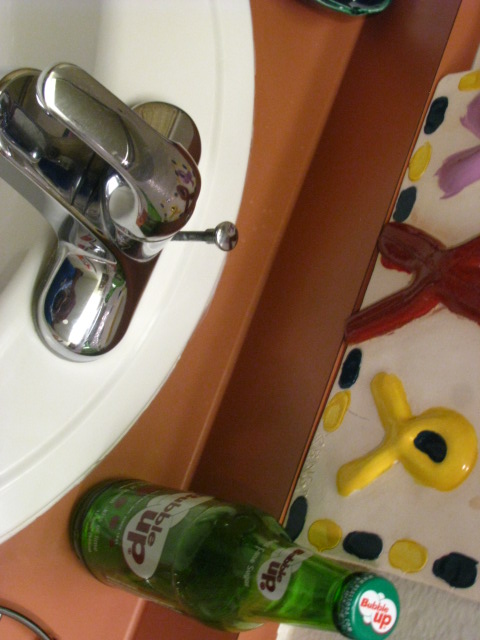This is an aerial close-up image of a child's bathroom sink. The sink is white and features a small, miniature water spout handle. The orange countertop provides a striking backdrop, contrasting with a child's painting mounted on the wall. The painting features vibrant colors, including yellow, red, purple, and black, and appears to be created with thick, dried paint on a white backdrop. Alongside the sink rests a transparent green soda bottle labeled "Bubble Up." The bottle has a green cap and features illustrations of bubbles, with "Bubble Up" written in red text on the bottle’s body and cap. The scene is set against a white wall, creating a colorful and lively yet orderly arrangement.